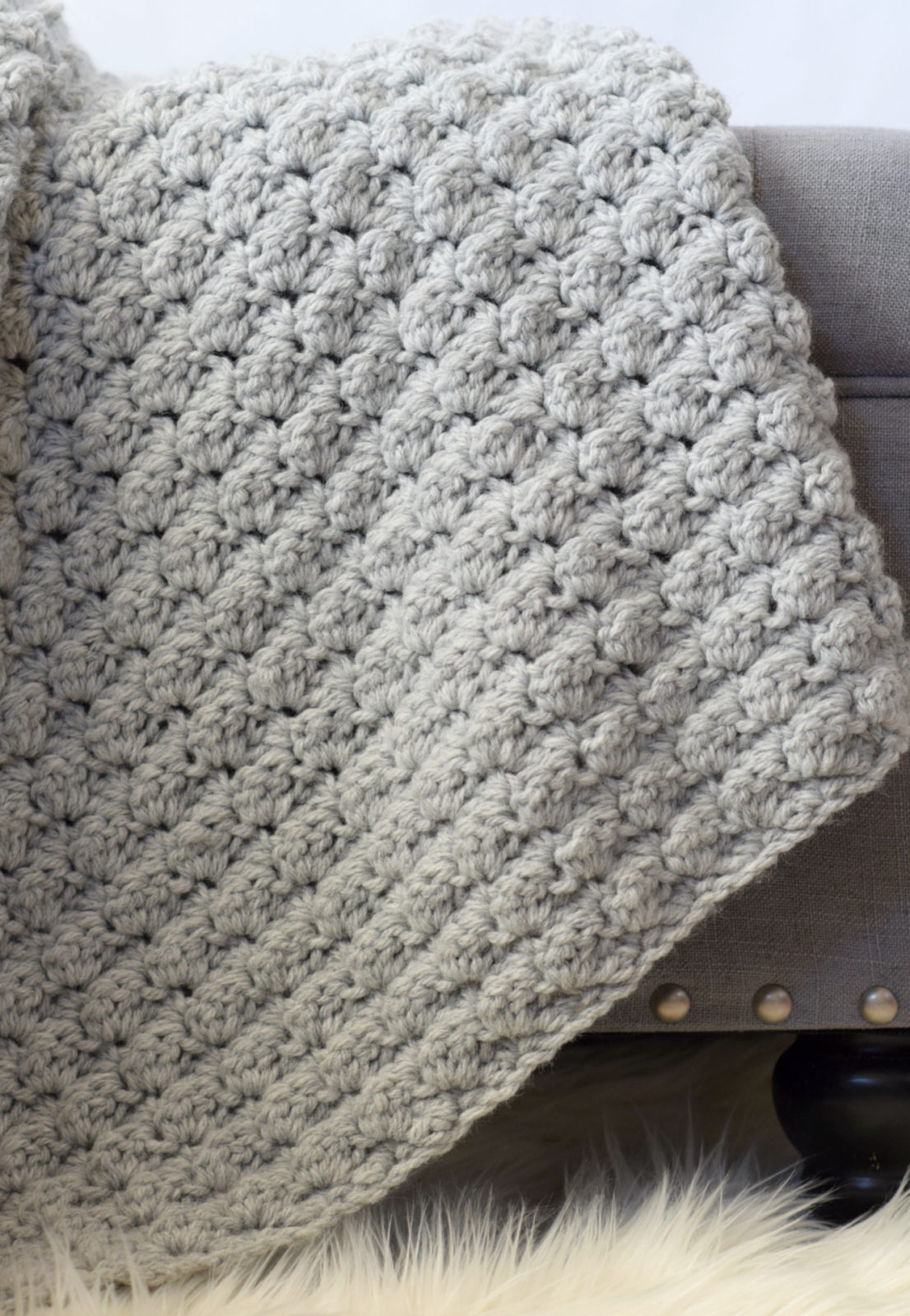The image captures a close-up view of a gray piece of furniture, likely a couch or chair, against a light blue wall backdrop that occupies a small portion of the top section. Dominating the scene is a large, light gray, wool-textured blanket, possibly crocheted, that appears soft and cozy. This blanket, covering approximately 80-90% of the furniture, drapes elegantly across it. Below the blanket, there's a feathery, white texture that is somewhat ambiguous—it could either be a fluffy white carpet or an animal, blending seamlessly with the overall gray and white color scheme. The furniture rests on a wooden floor, and the bottom-right corner features a black, peg-like leg of the sofa, accentuated by three little silver buttons. The overall focus is on the blanket, lending a sense of homeliness and comfort to the image.